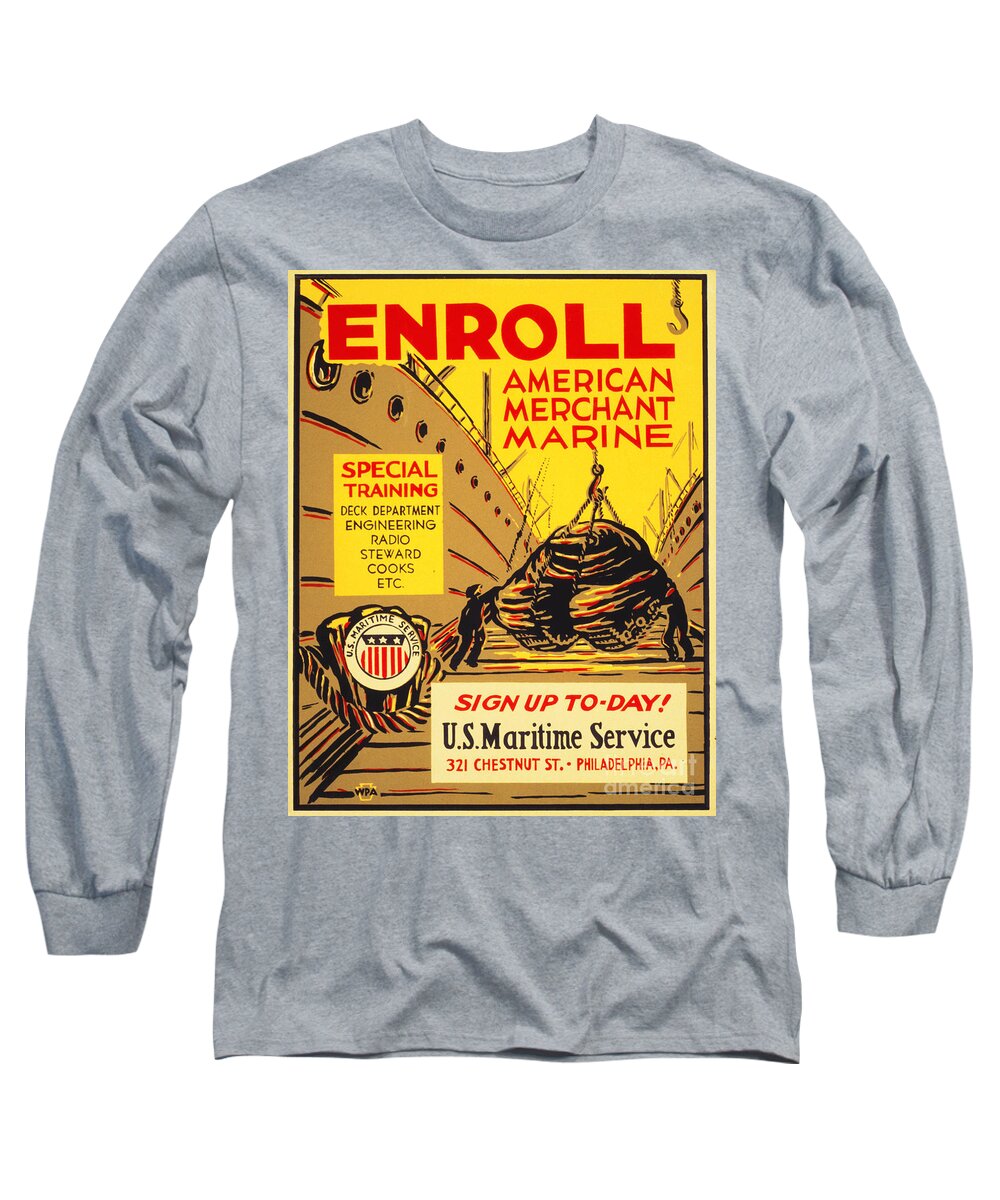In this image, we see a long-sleeved gray t-shirt laid against a white background. The t-shirt prominently features a graphic design in the center, resembling a vintage poster with a yellow base and comic-style drawing. The design includes an illustration of a dock scene, with a boat on one side and a bundle being hoisted down onto the dock by a crane, accompanied by figures in black silhouettes. At the top of the graphic, bold red letters spell out "ENROLL," followed by smaller red text reading "American Merchant Marine." On the left side of the image, a label in red text says "Special Training," with further details such as "Neck Department, Engineering, Radio, Steward, Cooks, etc." beneath it in black. On the right side, there is a smaller yellow box overlaid on the ship, labeled "special training." At the bottom of the graphic, a white box contains two lines: "Sign Up Today!" in red text and "US Maritime Service" in black, followed by "321 Chestnut Street, Philadelphia, PA" in smaller red text. The overall design elements and text evoke a sense of historical recruitment appeal, amplifying the t-shirt's vintage aesthetic.